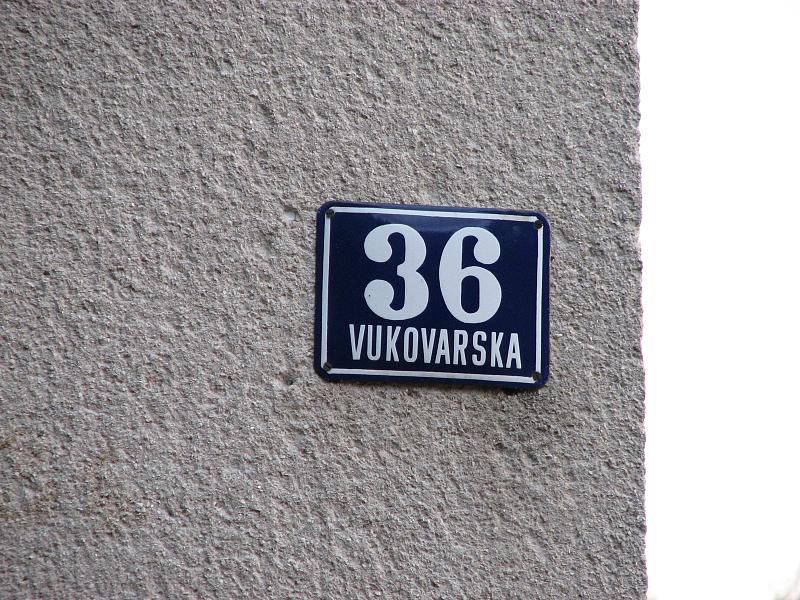In this color photo, a slightly tilted blue metallic plaque is mounted on a grayish-white concrete wall, likely part of a building. The plaque features a white-bordered edge and is secured with screws visible at each corner. Dominating the sign is the large, white number "36," followed below by the word "VUKOVARSKA" in white lettering. The gray concrete background suggests an exterior setting, though the exact location and purpose of the sign—perhaps indicating an address or parking spot—remain open to interpretation.